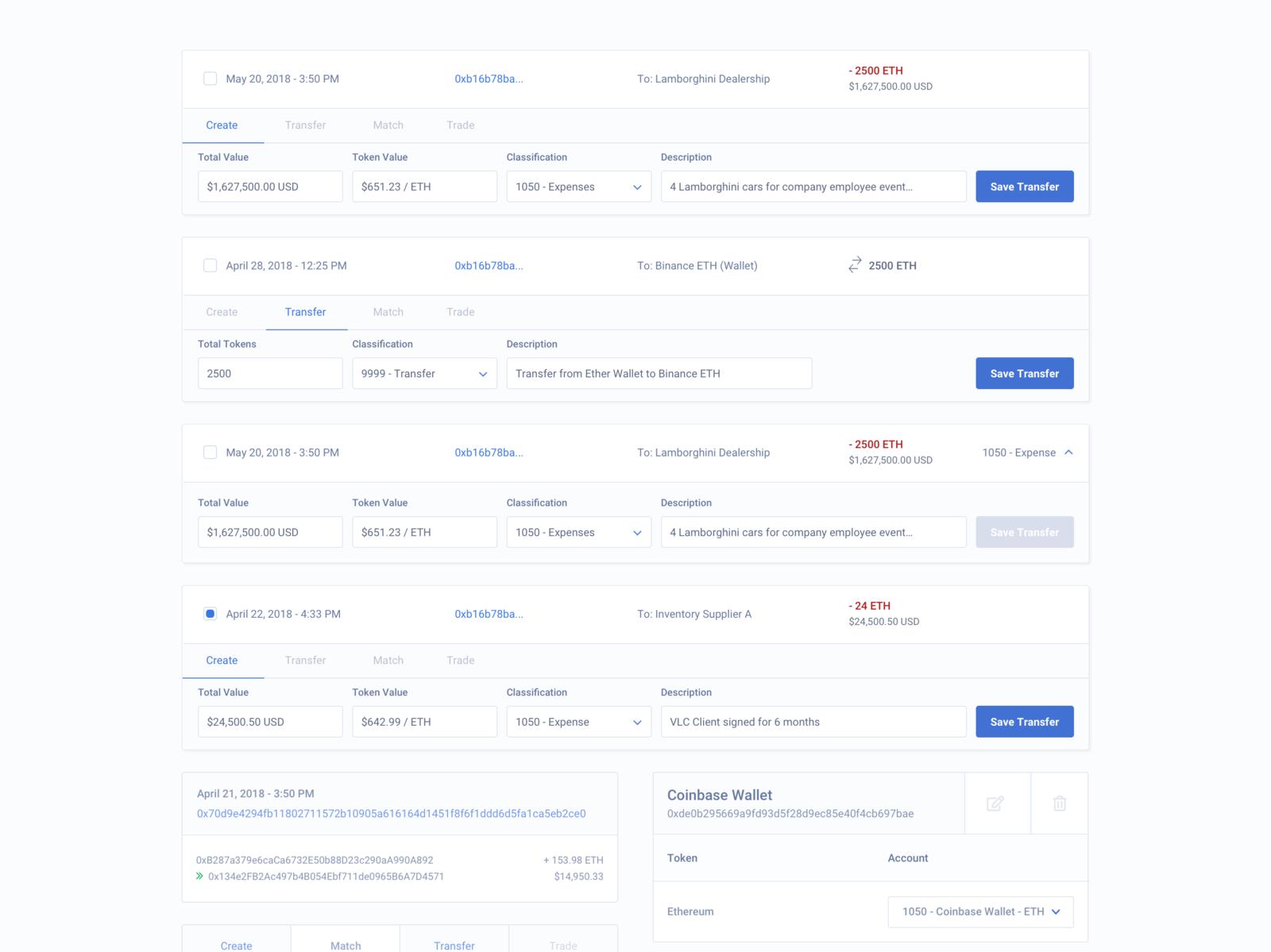**Descriptive Caption:**

This screenshot displays an interface of an organizational webpage or app featuring various entries in a clean and minimalistic design, characterized by a white background with blue accents. The layout includes four main entries, each encapsulated in rectangular boxes, sorted chronologically and containing crucial details such as dates, times, codes (possibly passwords), and destinations. Here's a detailed breakdown of the entries from top to bottom:

1. **First Entry**:
   - **Destination**: Lamborghini Dealership
   - Labeled with a date and time, a unique code, and relevant information.
   
2. **Second Entry**:
   - **Destination**: Finance ETH Wallet
   - Follows the same structured format with corresponding details.
   
3. **Third Entry**:
   - **Destination**: Lamborghini Dealership
   - Similar details as previous entries, featuring a unique code and specific date and time.
   
4. **Fourth Entry**:
   - **Destination**: Inventory Supplier A
   - Contains designated date, time, and other relevant information.

On closer inspection, the assumed fifth entry is actually two distinct sections. The left section provides a date and time, but lacks the comprehensive details found in the main entries. Adjacent to this, on the right, is a section labeled "Coinbase Wallet."

Additionally, the interface includes interactive tabs labeled "Create," "Transfer," "Match," and "Trade," along with a "Save Transfer" button. Notably, the "Save Transfer" button in the third entry from the top is grayed out, indicating unavailability or in-progress status for that particular entry.

Overall, the organized structure and minimalist design make navigation and interaction straightforward and efficient.